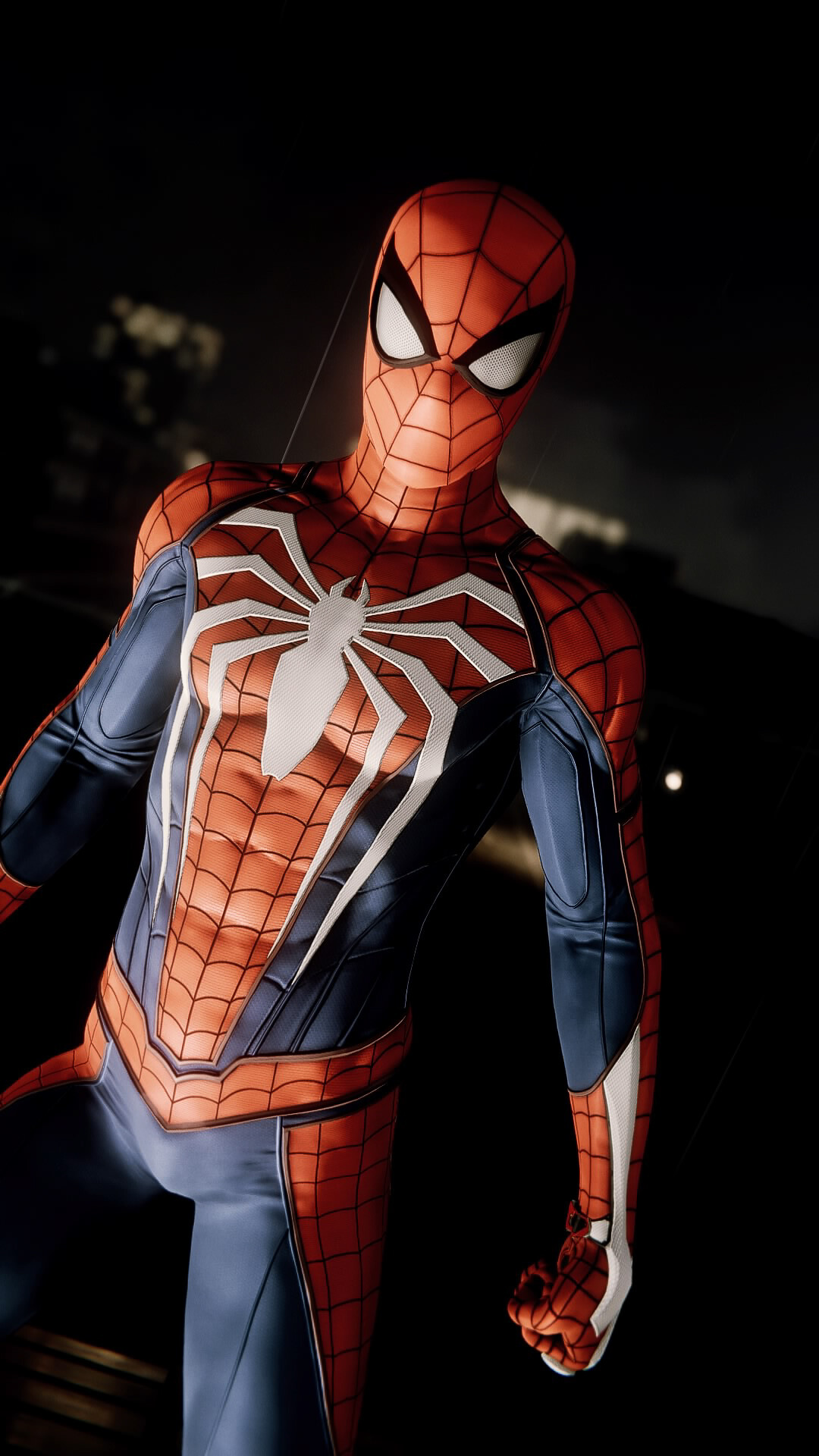This graphic animated 3D image depicts Spider-Man in his iconic red suit, featuring a prominent large white spider emblem on his chest. The spider's legs extend upward to his shoulders and downward to his waist. The inner sides of his arms are blue, with white accents running down to the backs of his hands. A web-like string trails behind him, adding dynamism to the scene. The background illuminates urban buildings, enhancing the action-packed atmosphere. Additional details include red accents around the back of his thighs and a white dot on his left arm. The suit also features padded areas emphasizing his muscular build.